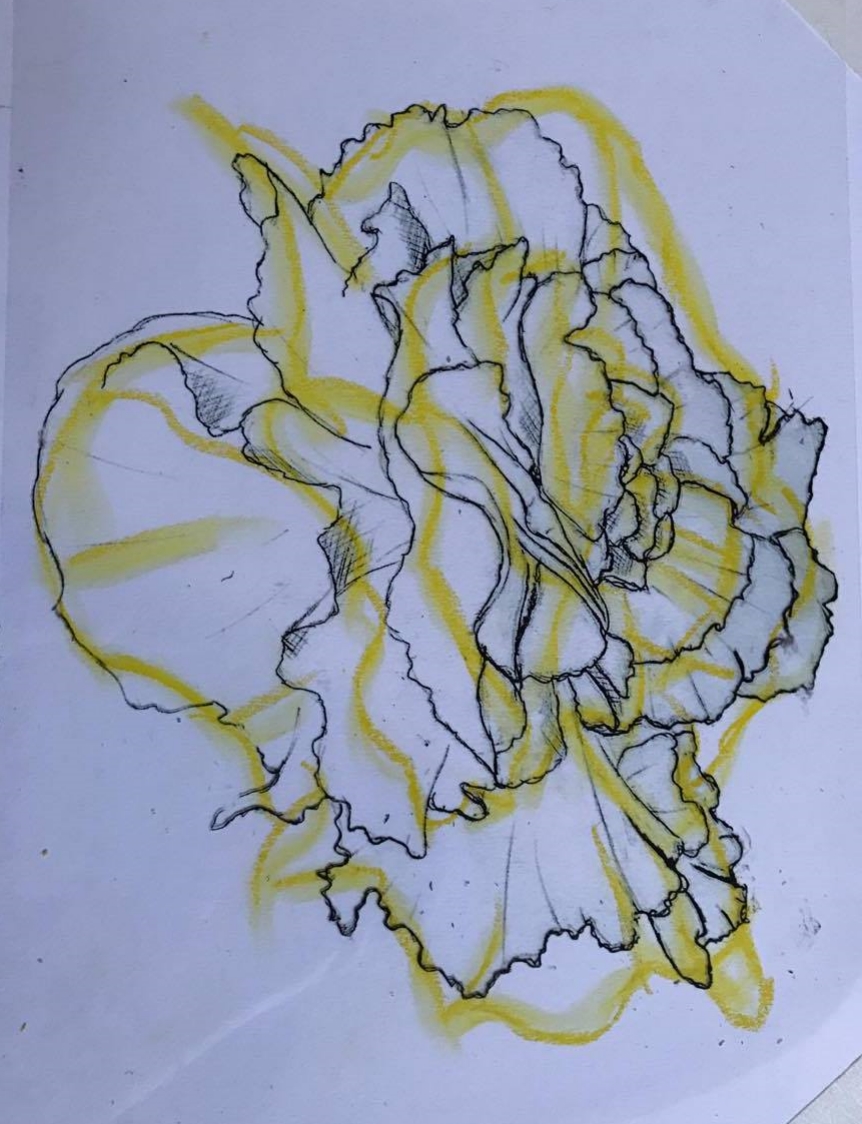The image features a detailed sketched drawing, possibly made with a black pencil or fine-tipped pen, of a flower against an off-white piece of paper with a blue hue, likely due to lighting. The drawing spans roughly one and a half to two times taller than it is wide, and the paper appears to be slightly tilted, with visible edges in the upper and lower right corners. The flower, which faces around the two to three o'clock position, showcases intricate details including lines, creases, and subtle shading on some petals, giving it a dimensional appearance. Over this precise sketch, a yellow marker has been used to trace around many of the major edges of the flower, adding a bright, almost golden hue accentuating the ridges. The overall result is a combination of meticulous black line work and playful yellow highlights that enhance the floral structure.